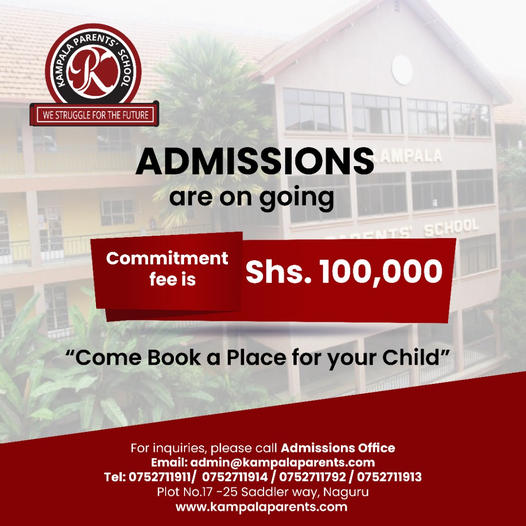The advertisement for Karpala Parents School, prominently displays the school's round logo, featuring a striking combination of red, black, and white colors. Beneath the logo, the motto "We struggle for the future" is clearly visible, emphasizing the school's commitment to educational excellence.

The main body of the advertisement announces that admissions are currently open, with a commitment fee set at SH 100,000. A parenthetical note invites prospective parents to "come book a place for your child," encouraging early enrollment.

At the bottom of the advertisement, contact information is provided for further inquiries. Prospective parents can reach the admissions office via email at admin@karpalaparents.com or by calling any of the following telephone numbers: 0752711911, 0752711914, 0752711792, or 0752711913.

The advertisement also lists the school's location at Plot Number 17-25, Sadler Way, Niagara, and directs interested individuals to visit their website at karpalaparents.com for more information.

The background of the advertisement features a faint image of a school building that closely resembles a house, set against a backdrop of peaceful trees, evoking a sense of a serene and nurturing educational environment.